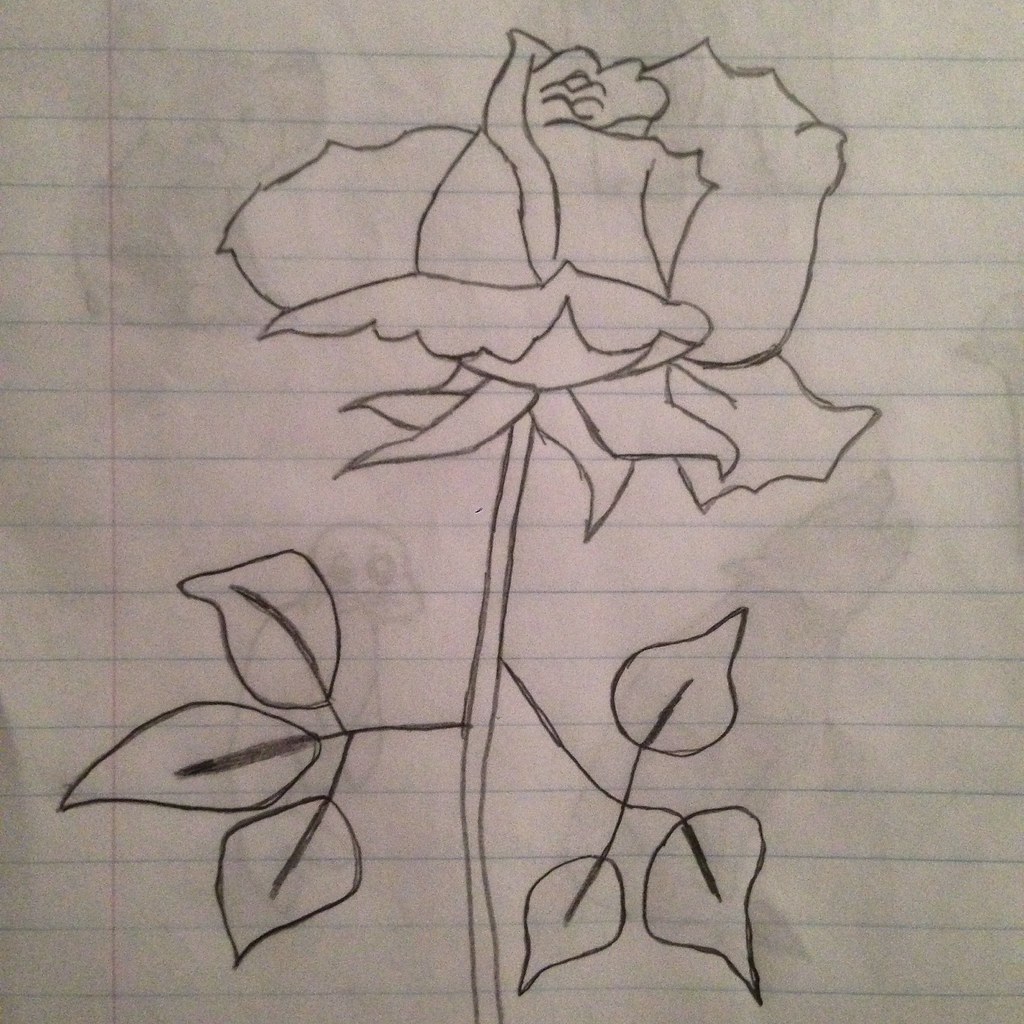A detailed hand-drawn sketch of a rose on a standard piece of notebook paper with blue horizontal lines and a lightly colored red vertical margin on the left. The pencil drawing features a single rose with a stem rising from the bottom of the page. About two-thirds up, the stem splits into two smaller branches, each adorned with three intricately detailed leaves, complete with visible central spines. The main rose bloom at the top has approximately six to seven petals, with the inner petals curled tightly while the outer petals are beginning to unfurl, suggesting they might soon fall off. Additionally, there are faint sketches of animals in the background—likely remnants from the next page of the notebook—including a koala, a bird, and a dog. These shadowy images add an intriguing, almost ghost-like element to the drawing but do not detract from the focus on the rose.